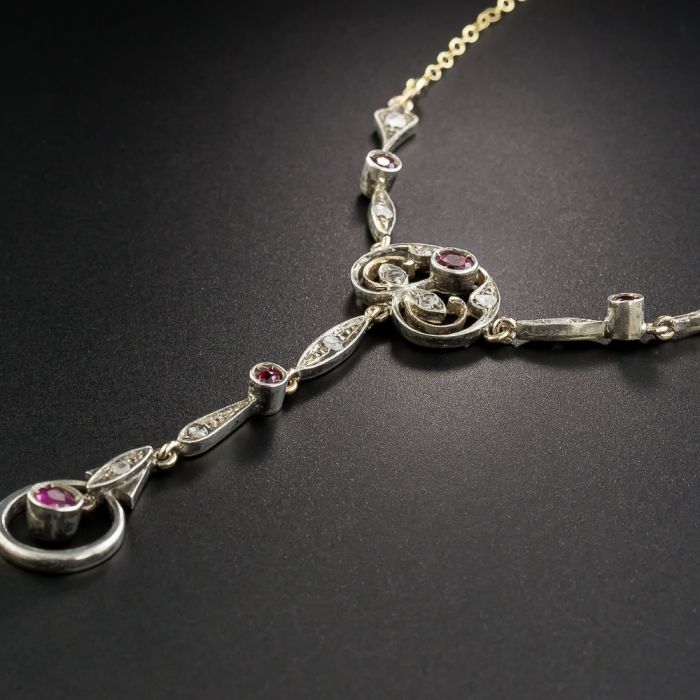The photograph is a vertically rectangular, almost square, color image of a staged close-up shot. The background is a dark gray or black surface, and the focus is on a long, elaborate necklace adorned with multiple stones and charms. The primary structure of the necklace combines both gold and silver chains, with several distinct decorative elements.

Starting from the bottom, there is a prominent purple stone that catches the light, making it appear shiny but dark. A few chains up, there's a cylindrical silver element set with another purple or reddish stone. This portion extends into a heart or oval-shaped section adorned with red stones and diamond-like embellishments, which serves as the main ornament.

Hanging from this central piece are two extensions, each terminating in leaf-shaped charms encrusted with diamonds. Notably, the upper part of the necklace features a red stone framed by diamond-like settings, contributing to the central, eye-catching motif. The photograph is brightly lit from an artificial light source, illuminating the upper portion more than the lower, and the necklace is presented slightly sideways, resembling the outline of a key.